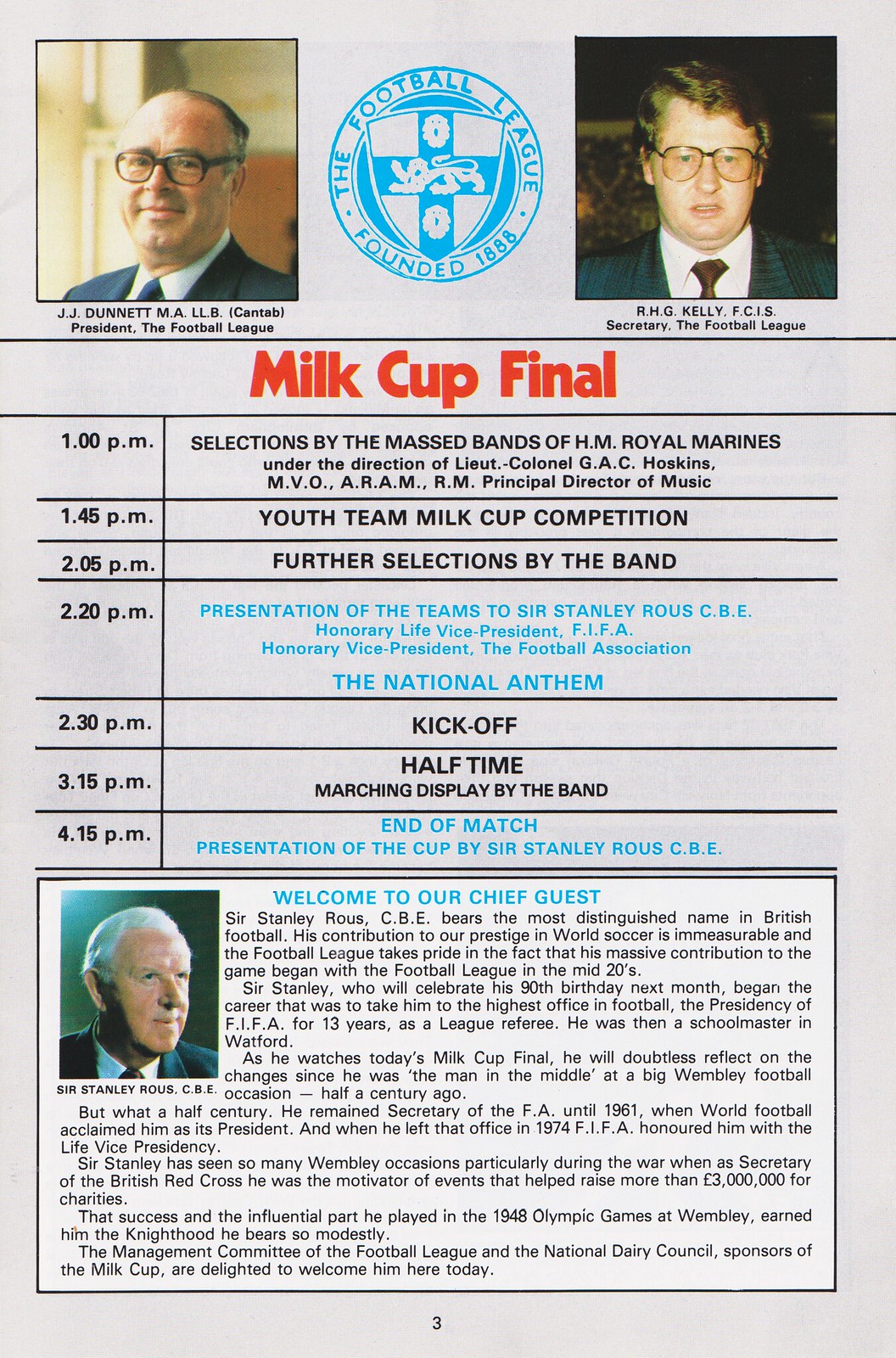This detailed digital poster for the "Milk Cup Final" event features a comprehensive layout on a light gray background. At the top center, a prominent blue logo of a football league founded in 1888 is flanked by photographs of two men on either side—one in the top left and the other in the top right corner. Each photograph includes the individual's name and details beneath them. Below the logo, the event title "Milk Cup Final" is written in bold red. A black line runs horizontally beneath this title, followed by a schedule with timings on the left and corresponding event details on the right. The text of the schedule is in black, with the fourth and seventh entries highlighted in blue. Lower down, a white box contains the title "Welcome to Our Chief Guest" in blue, along with a photograph of a man from the neck up situated at the top left of the box, and additional text taking up the rest of the space. The overall design is structured to provide clear information about timelines and key individuals involved in the event, with a well-organized and visually coherent presentation.